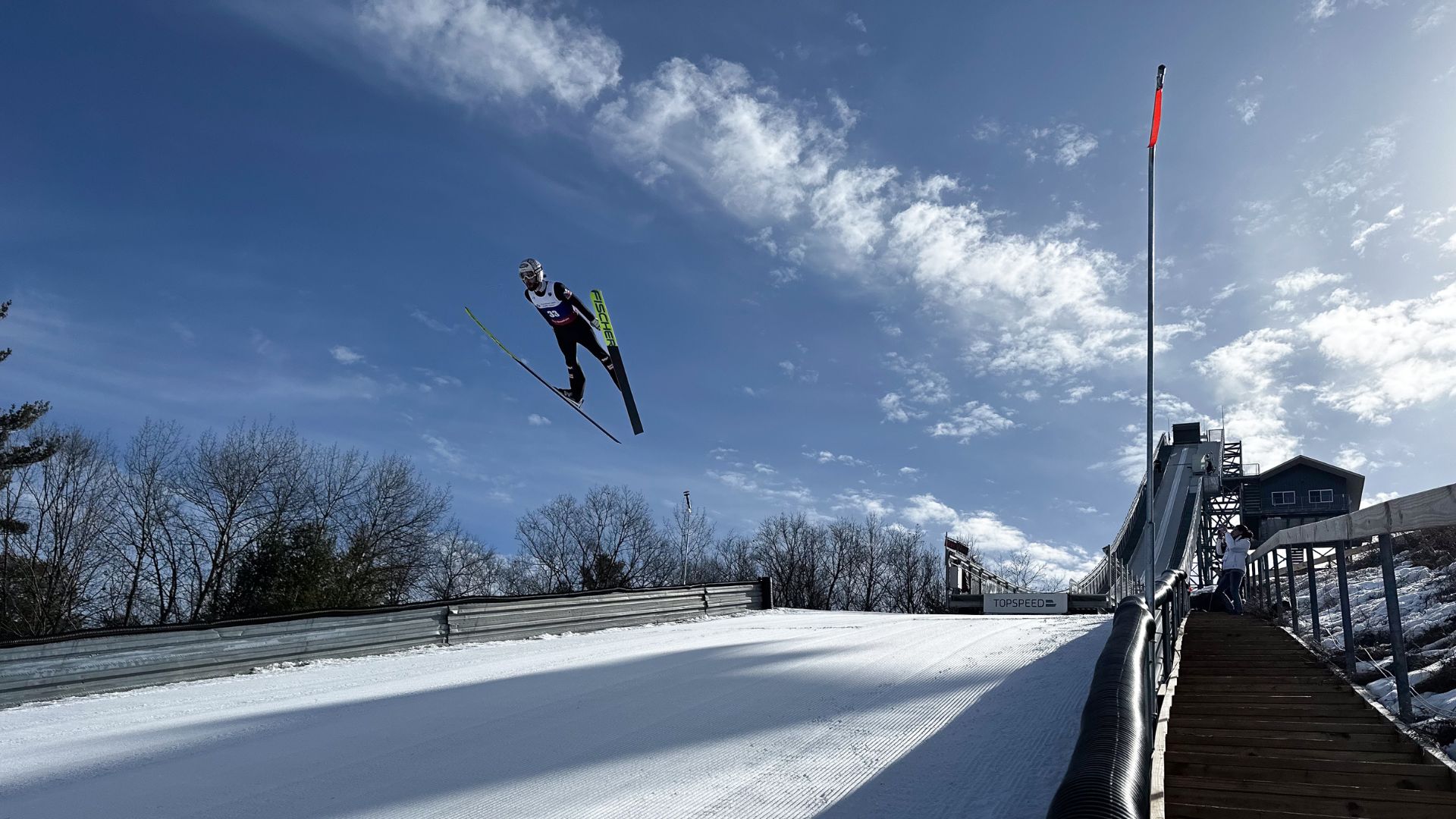The photograph captures a thrilling moment at a ski resort, showcasing an exhilarating ski jump on a snowy, cloud-covered daytime. A skier, attired in a white and blue shirt and black ski pants, is airborne, executing a spectacular jump with their skis fanned out—one clearly visible with blue and yellow hues. The skier is equipped with headgear and speed goggles, emphasizing their high-speed descent. To the right of the scene, a woman in a white winter jacket and blue pants stands on the ski slope's walkway, capturing the action with her camera. The ski slope itself is lined with trees on the left and features a small ski shack with two windows on the right. At the top of the ramp—the point of the skier's launch—there is a gray-lined railing, with the phrase "top speed" marked at the launching base, highlighting the intense nature of the jump.